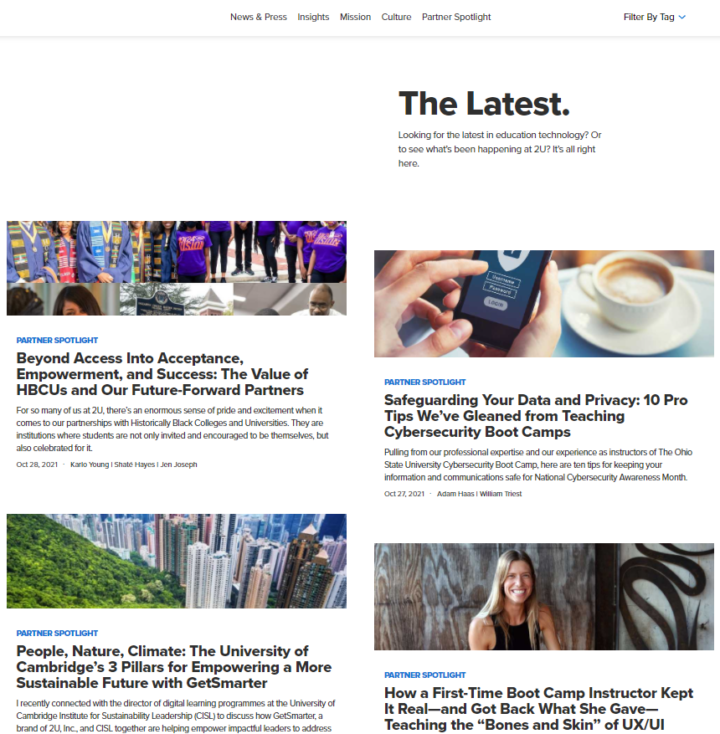The screenshot is in portrait mode, showcasing a user interface with several tab headings centered at the top. These tabs are labeled: "News and Press," "Insights," "Mission," "Culture," and "Partner Spotlight." In the upper right-hand corner, there's an option labeled "Filter by Tag" with a blue drop-down arrow next to it. Directly beneath these elements is a gray stripe stretching across.

The main content area is prominently white and begins with a bold heading, "The Latest." Below this heading, a subheader reads: "Looking for the latest in education technology or to see what's been happening at 2U? It's all right here."

The content area is divided into four sections, each featuring an image, article title, and link, although the layout seems somewhat imbalanced. 

1. **Top Left Section:**
   - An amalgamation of multiple images under the heading "Partner Spotlight" in blue.
   - The article titled "Beyond Access into Acceptance, Empowerment, and Access: The Value of HBCUs and Our Future Forward Partners" is available for click-through.

2. **Top Right Section:**
   - An image depicting a person using a cellphone next to a cup of coffee.
   - The article is titled "Safeguarding Your Data and Privacy: 10 Pro Tips We Gleaned from Teaching Cybersecurity Boot Camps."

3. **Bottom Left Section:**
   - An image showcasing a lush green area juxtaposed with a cityscape.
   - The article is titled "People, Nature, Climate: The University of Cambridge's Three Pillars for Empowering a More Sustainable Future with GetSmarter."

4. **Bottom Right Section:**
   - Featured is an article titled "How a First-Time Boot Camp Instructor Kept It Real." However, no specific image description is provided.

Each section corresponds to specific topics within the broader themes of education technology and institutional initiatives, providing clickable links for further reading.